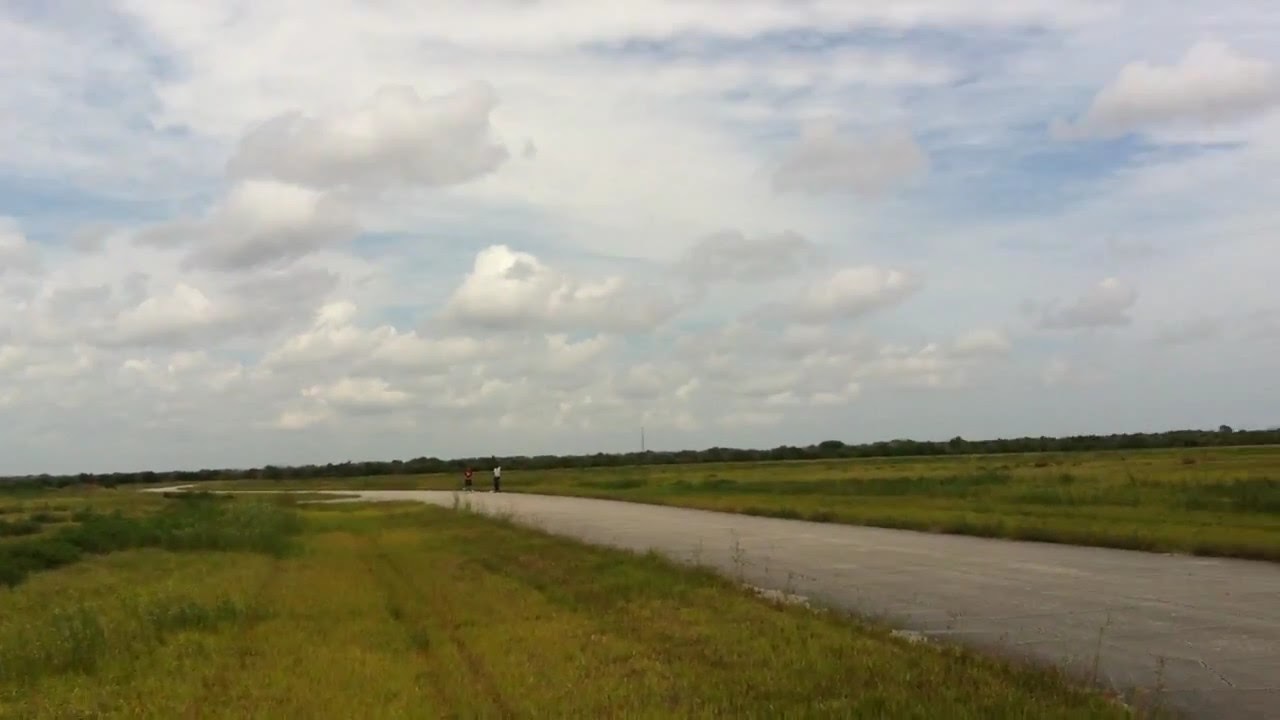A photograph captures a serene rural scene dominated by a paved country road stretching from the bottom right corner and curving gently to the left before disappearing into the horizon. On either side, expansive fields of grasses extend up to the distant horizon, where a line of trees spans from the left to the right. The sky above is light blue, dotted with fluffy white clouds, occupying about two-thirds of the frame. In the middle distance, slightly left of center and close to an apparent intersection, two people can be seen walking along the road. One individual is dressed in a white top and black pants, while the other wears dark pants and possibly a red top, although the distance makes it hard to discern. This tranquil setting evokes a sense of peace and simplicity, characteristic of a countryside or farmland environment.